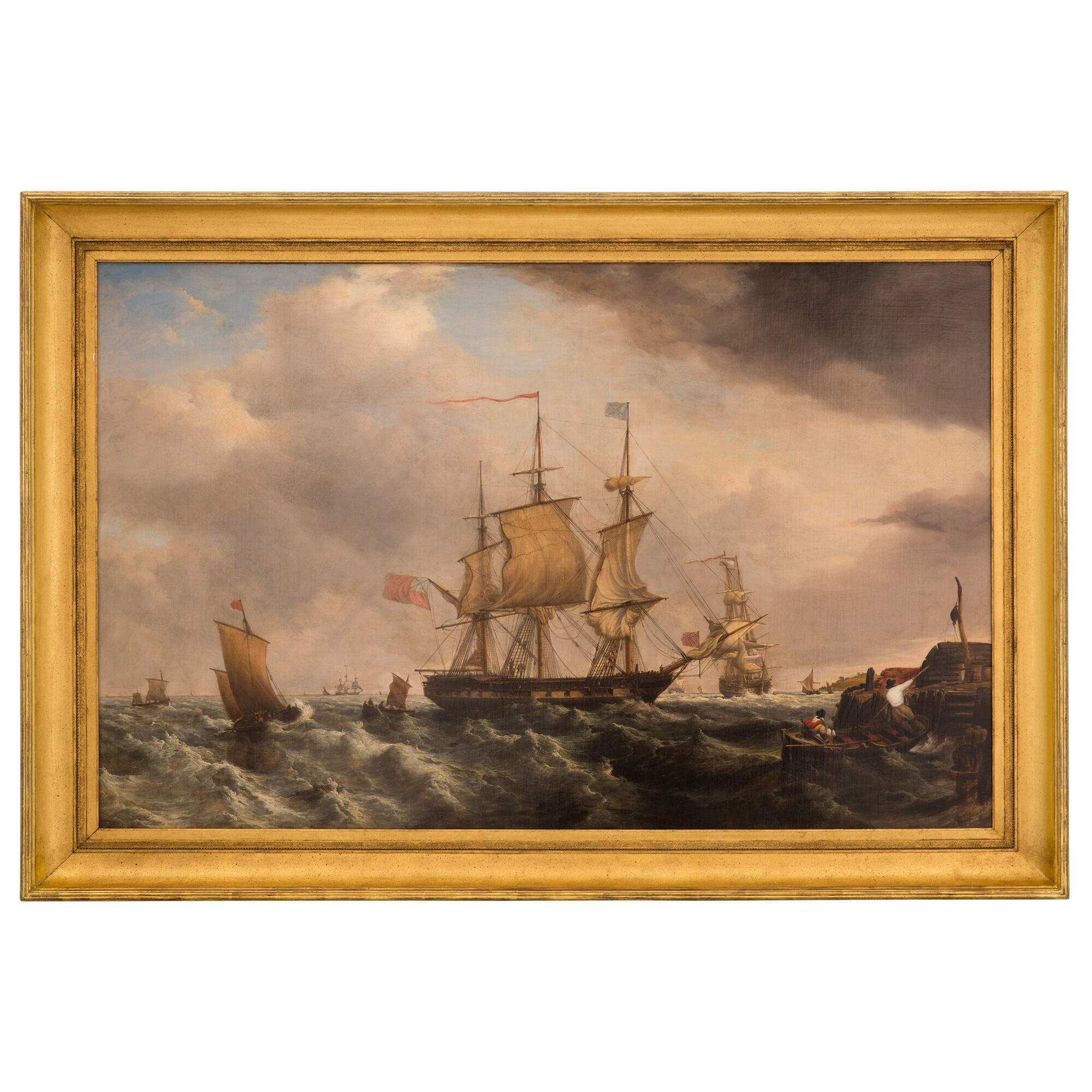This is a photograph of an older oil painting, set in a gold frame, depicting a dramatic maritime scene. Central to the image is a large schooner with billowing white sails, prominently marked by a long, thin red flag and a smaller light blue flag blowing in the wind. The ship navigates rough, choppy waters with white-capped waves amid a backdrop of ominous dark clouds on the right and contrasting puffy white clouds and patches of blue sky on the left. Surrounding the main vessel are several smaller ships, also caught in the treacherous seas. The overall ambiance of the painting evokes a sense of peril and a subtle pirate vibe, emphasizing the danger and uncertainty of the ocean voyage.